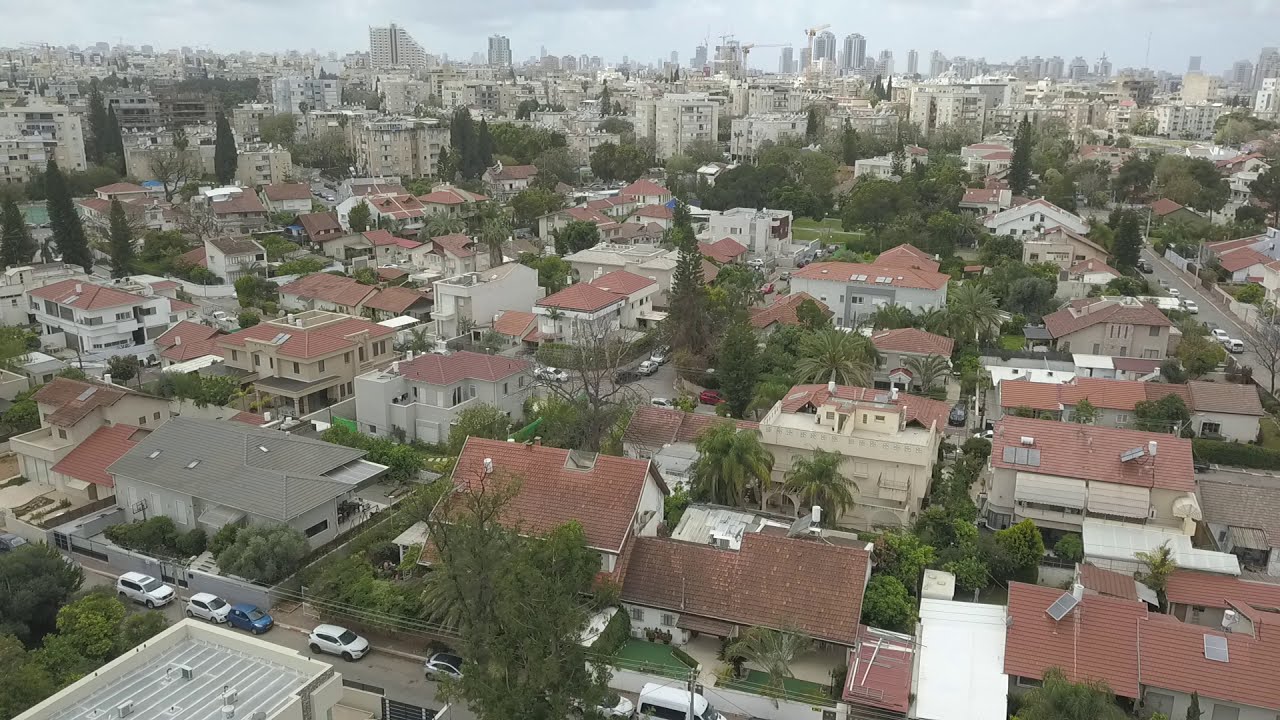The photograph captures an aerial view of a densely populated European city with a harmonious blend of residential and commercial zones. The foreground reveals a bustling neighborhood characterized by multi-story residential buildings with distinctive red tiled roofs, some equipped with solar panels, and a mix of gray and beige façades. Interspersed throughout are tree-lined, two-lane streets, including notable palm trees contributing green to the concrete setting. As the view extends towards the horizon, the buildings rise in stature, transitioning into a skyline dominated by imposing skyscrapers and active construction cranes, constructing even taller structures. The cityscape is bathed in daylight, under a gray-blue sky, emphasizing the intense urban development and the city's vibrant, somewhat overwhelming, architectural footprint.